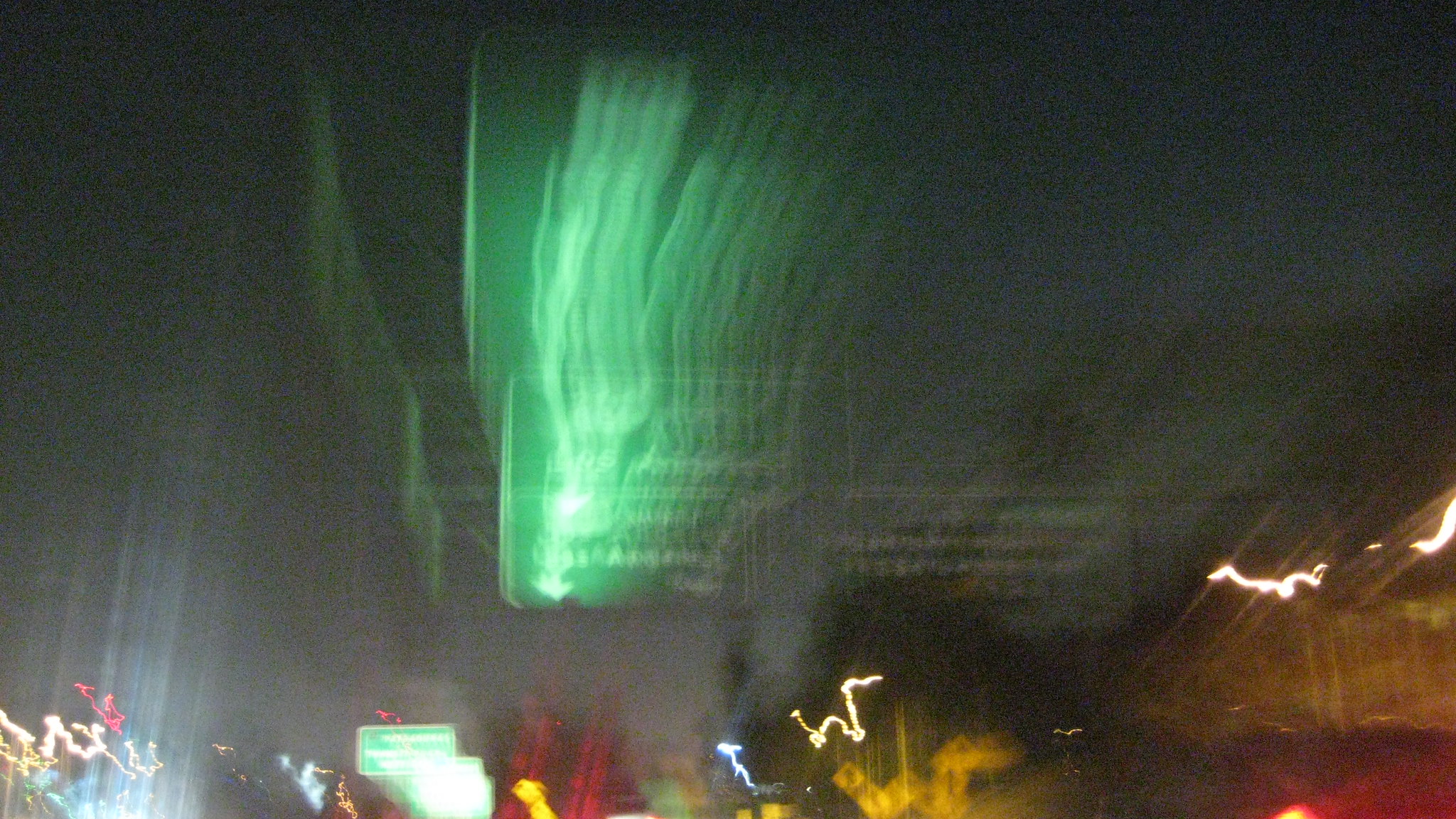In this nighttime image, a blurred green rectangular light streaks upwards through the dark sky, adding an air of mystery. The background is dominated by a large white rectangular structure, possibly a building, that stands prominently against the night. At the bottom of the horizontal image, a variety of bright, colorful lights in reds, yellows, and whites illuminate the scene, likely from streetlights and city signage. Among these lights, a street sign and an unreadable road sign are visible, possibly indicating directions to Los Angeles. Interestingly, the street sign appears duplicated at the center of the image, contributing to the blurred and chaotic ambiance of the photograph.